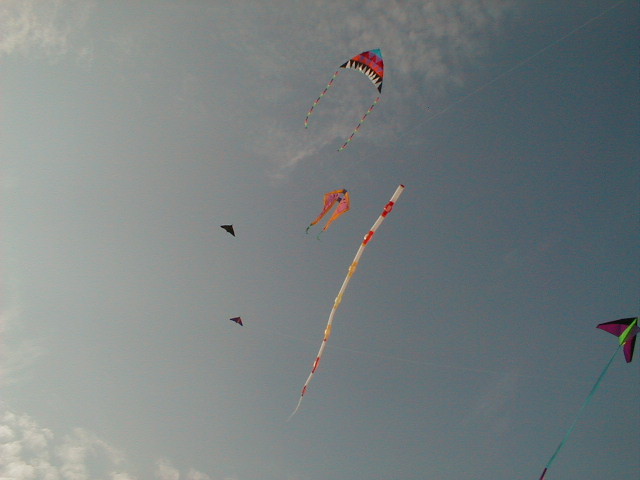This vivid outdoor photograph captures a mesmerizing view of the sky adorned with a plethora of kites. The sky ranges from a deep blue on the right to a lighter blue with wispy, diffuse clouds scattered throughout. From the underneath perspective, the image showcases a vibrant display of kites of various shapes and sizes. Dominating the sky, there is a long, snake-like kite featuring alternating shades of red, orange, yellow, and white. Another striking kite displays a complex pattern with a blue tip, followed by sections of red, black, and white, accompanied by two multicolored streamers flowing from each side. Smaller, triangular black kites add contrast, appearing either farther away or simply dark. On the bottom right, a distinctive pink, green, and black triangular kite with a turquoise tail can be partially seen. This lively tableau of kites against the dynamic backdrop of the sky and clouds creates a captivating and cheerful scene.